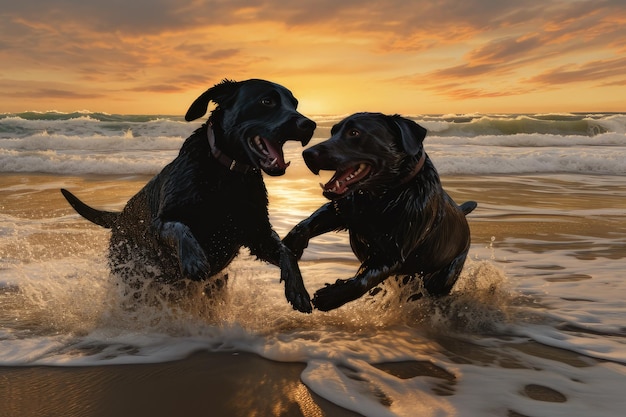This vibrant, lifelike painting captures two playful black Labrador Retrievers in mid-action on a sandy beach, with their mouths open and ears flapping. The dogs, appearing to wrestle or leap in a joyous frolic, are surrounded by splashing water as the waves lap at their feet and break into white and green bubbles around them. Narrow tails extend outward, evidence of their high-spirited romp. The background features a horizon where the ocean meets the sky, painted with an array of sunset or dawn hues—deep reds, glowing oranges, and light yellows. Partly cloudy, the sky casts a magical twilight tint over the scene, highlighting the happy, carefree energy of the moment.